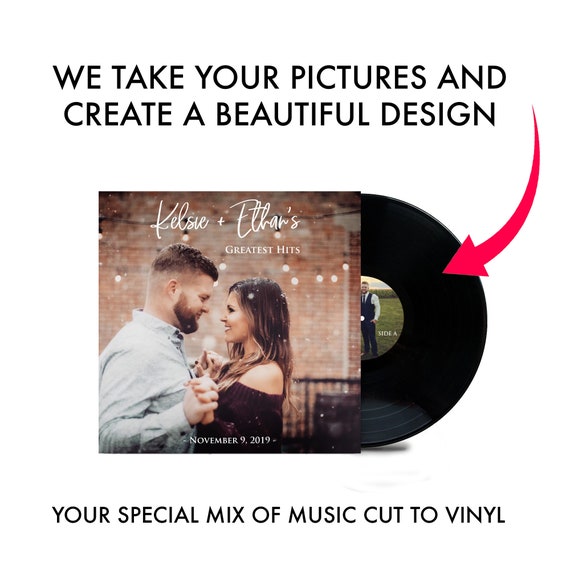This advertisement showcases a service that transforms your cherished photos into beautiful vinyl record designs. Set against a white background, the ad features bold black text at the top: "We take your pictures and create a beautiful design." Central to the image is a vinyl record halfway out of its custom-designed sleeve. The sleeve itself displays a charming photograph of a couple, Kelsey and Ethan, gazing lovingly into each other’s eyes while holding hands, standing in front of a brick wall adorned with outdoor string lights. Above the couple in white text, it reads "Kelsey and Ethan's Greatest Hits," with the significant date "November 9th, 2019" below them. A red arrow points to the vinyl record, which features a smaller picture of the couple in its center and is labeled "Side A." At the bottom of the ad, in black text, it says, "Your special mix of music cut to vinyl."